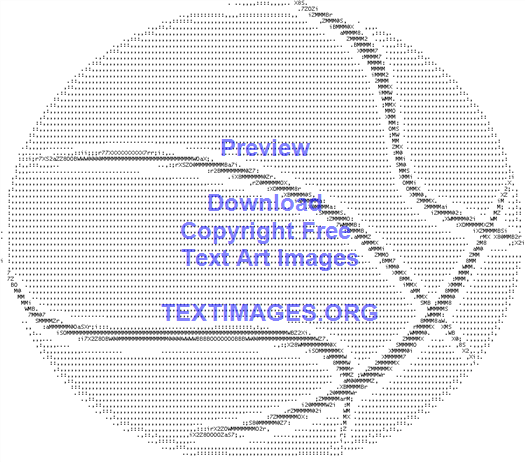The image depicts a black and white graphic resembling a basketball, created entirely from text characters. The basketball shape is detailed with dark gray lines and numerous tiny black dots, giving it the appearance of having been made with a typewriter. At the center of this text art is a prominent section of blue text. The blue text is centered and reads, in order, "PREVIEW," followed by "DOWNLOAD COPYRIGHT FREE TEXT ART IMAGES," and in larger capital letters, "TEXTIMAGES.ORG." The combination of the detailed text-based basketball graphic and the centrally-placed blue informational text suggests there was an issue with the image, possibly indicating it's a sample or placeholder from the website TextImages.org.